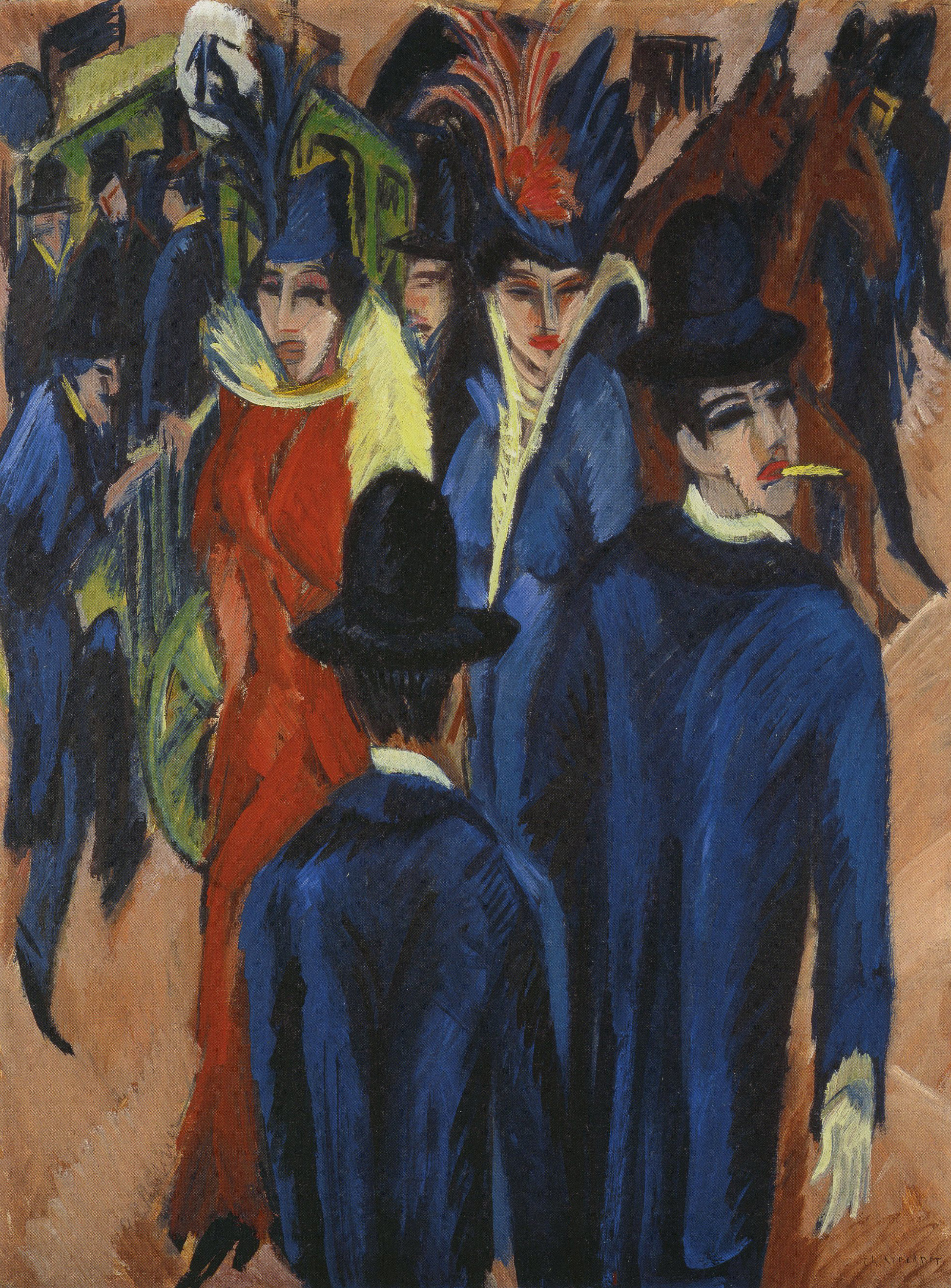This intricate, somewhat abstract painting depicts a group of affluent individuals at what appears to be an equestrian event. Standing out in the foreground are four meticulously dressed figures, likely couples, underscoring their wealth and social standing. The two gentlemen are both attired in distinctive blue suits and black hats; one faces us with a cigarette, while the other has his back turned. The two elegantly adorned women wear detailed gowns, one in vibrant blue and the other in striking red. They don extravagant feathered hats and furs, their expressions almost surreal and stylized. The background features additional figures, mostly men in blue coats and hats, and includes two noticeable brown horses possibly being guided by a policeman. The painting employs a varied palette of black, white, gray, shades of blue, yellow, red, brown, green, and gold, set against a light tan background, enriching the visual complexity and historical ambiance of the scene.